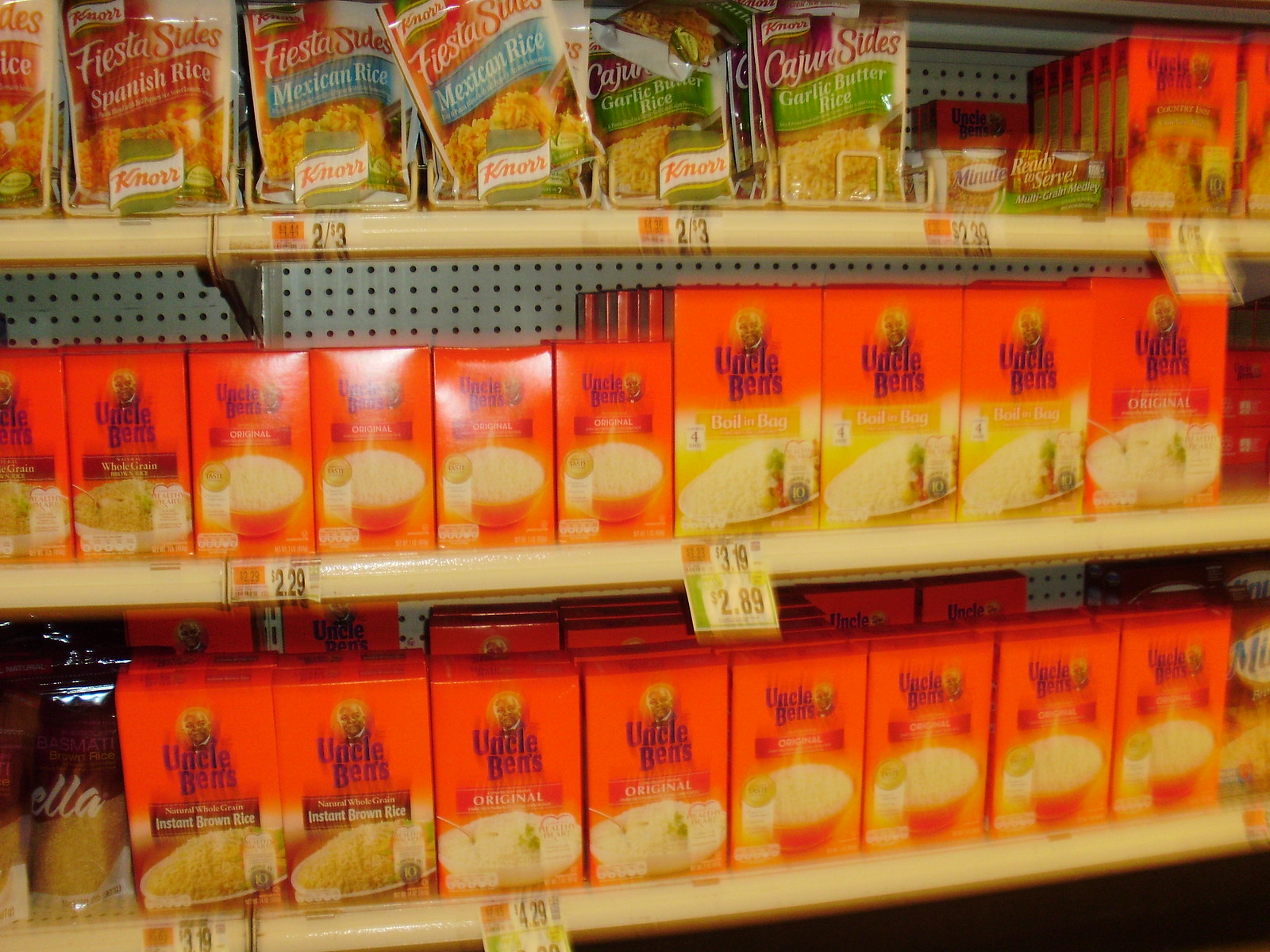This photograph, although slightly blurred, captures three well-stocked shelves in a grocery store's grain and pasta aisle, predominantly featuring various types of rice, with a notable emphasis on Uncle Ben's products. The top shelf displays an array of rice bags, including brands like Knorr and Fiesta Sides, offering varieties such as Spanish Rice, Mexican Rice, and Garlic Butter Rice. There's also Minute Rice positioned to the right. The middle shelf is filled with bright orange Uncle Ben's rice boxes, neatly arranged with smaller boxes on the left and larger boxes on the right. These include a mix of white grain, whole grain, and boil-in-the-bag options. The bottom shelf is almost entirely dedicated to Uncle Ben's smaller boxes, including both original and instant brown rice flavors, lined up eight boxes across the front with multiple rows behind them. Each shelf has a price tag strip beneath it; the top shelf items are priced at two for three dollars, the middle shelf ranges from $2.29 for smaller boxes to $2.89 for larger ones, and the bottom shelf items are priced at $4.29. Despite some blurriness, the image faintly reveals a couple of non-Uncle Ben's products flanking the bottom row, potentially labeled as "Ella" or similar, adding diversity to the rice-centric display.